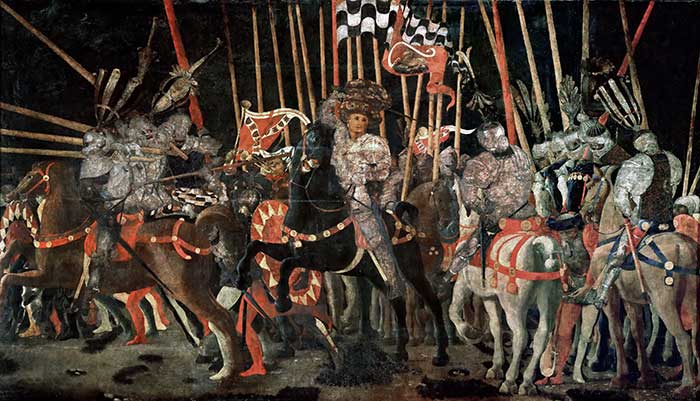The image, resembling a Renaissance painting, depicts a dramatic battle scene set against a dark background. The foreground is populated with an array of knights in gleaming silver armor, mounted on horses that vary in color from white to brown. These knights are equipped with long, elaborate arrangements extending from their hats. Central to the scene is a woman of apparent royalty, distinguished by her intricate white outfit and extravagant headdress. She is mounted on a rearing black steed, which is adorned with elaborate red and gold bridles and chest bands featuring ornate decorations. Surrounding her are other knights on their steeds, with each horse possessing decorative red straps and tassels, emphasizing the grandeur and tension of the moment. Behind the main action, wooden spears, poles, and black and white checkered flags rise into the darkened sky, adding to the historical and martial atmosphere. Some figures appear chalky, adding to the aged feel of the image, with one particularly disheveled man bound in red, evoking a sense of capture and struggle. Red and white pennants wave above the scene, providing a stark contrast against the dark backdrop.